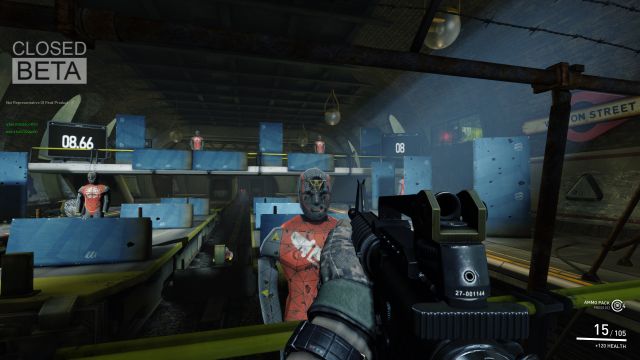The image depicts an industrial-themed area resembling a shooting or gun range, possibly within a video game environment. The scene is dominated by an ominous atmosphere, highlighted by a "CLOSED" sign in the top left corner, followed by "BETA" in bold black letters on a gray background, indicating it is a closed beta version of the game. To the back of this dark, industrial setting, shelves house what appear to be robot targets. These targets are progressively closer to the foreground, with one mere inches from the camera, revealing eerie, non-human facial features. In the forefront, a machine gun, held by a person visible only by their left hand and watch, is aimed directly at the closest target. The screen is overlaid with a HUD element displaying "8.66" over one of the figures, potentially a health or score indicator, reminiscent of classic first-person shooter games like Doom. Two gamers in grayish-red shirts are also visible, with one of them showing a health status of "15/105," adding to the realistic gaming interface and suspenseful setting.